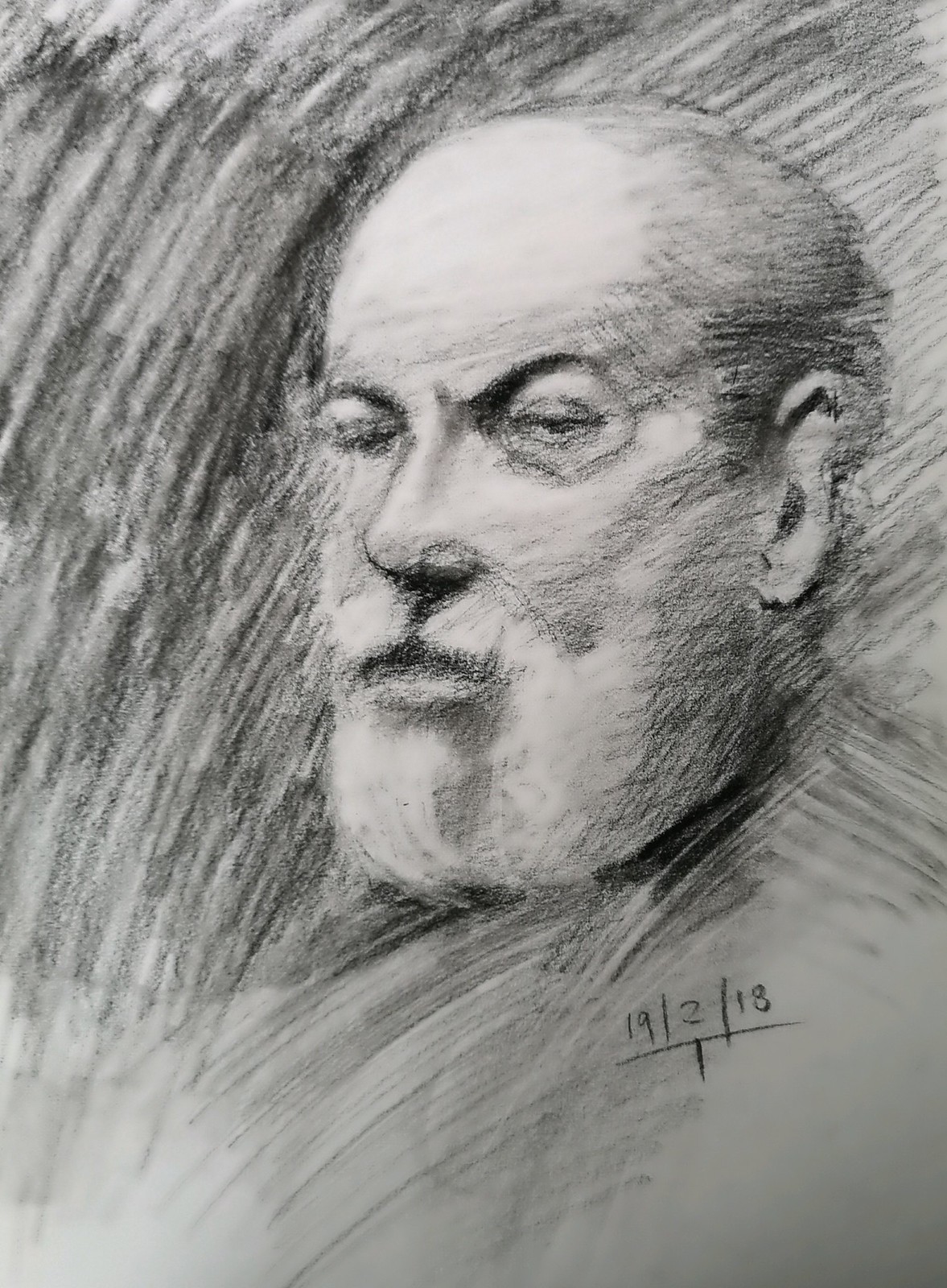This is a detailed pencil (possibly charcoal) sketch on a white piece of paper depicting an older man, potentially a self-portrait. The man appears to be balding with a closely-trimmed white beard and mustache. His facial expression conveys a serious or slightly intimidating demeanor, emphasized by his arched eyebrows. His head is skillfully shaded to stand out against the background, which is also meticulously darkened with pencil strokes. Notable facial features include his prominent right ear and partially visible left ear. He appears to be wearing a suit beneath his chin, adding a formal touch to the portrait. A date, 19-2-18, is inscribed at the lower part of the sketch, suggesting it was completed on February 18, 2019, or another date configuration, possibly accompanied by a faint "T."